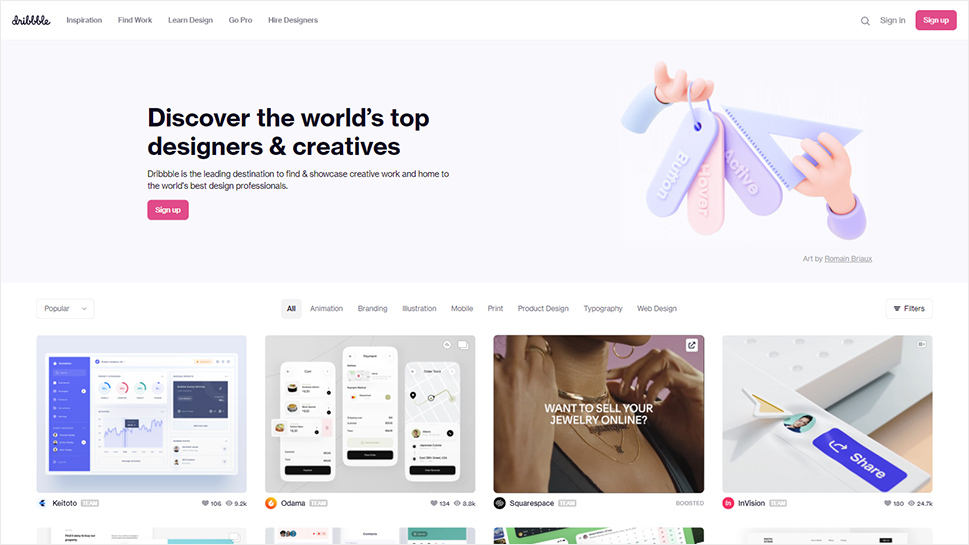**Caption:**

This screenshot captures the homepage of the Dribbble website, a leading platform for designers and creatives. In the top left corner, the Dribbble logo is elegantly displayed in lowercase cursive. Adjacent to the logo are several navigation tabs labeled "Integration," "Find Work," "Learn Design," "Go Pro," and "Hire Designers." On the top right, a magnifying glass icon signifies the search function, followed by "Sign In," and a prominent red "Sign Up" button with white text.

Centered on the page, a bold headline reads, “Discover the World's Top Designers and Creatives.” Beneath this headline, a descriptive paragraph in smaller font states, “Dribbble is the leading destination to find and showcase creative work and home to the world's best design professionals.” Directly below this text, another red "Sign Up" button with white text invites users to join the community.

To the right, a playful graphic showcases two cartoon-like hands; the left hand holds a ring of three tags labeled "Button," "Hover," and "Active," while the right hand features a purple protractor.

At the bottom center, additional navigation tabs such as "Animation," "Branding," and more can be seen. The page showcases various thumbnails of website designs and features, illustrating the diverse array of creative work available on the platform, catering to both creators and consumers interested in design.